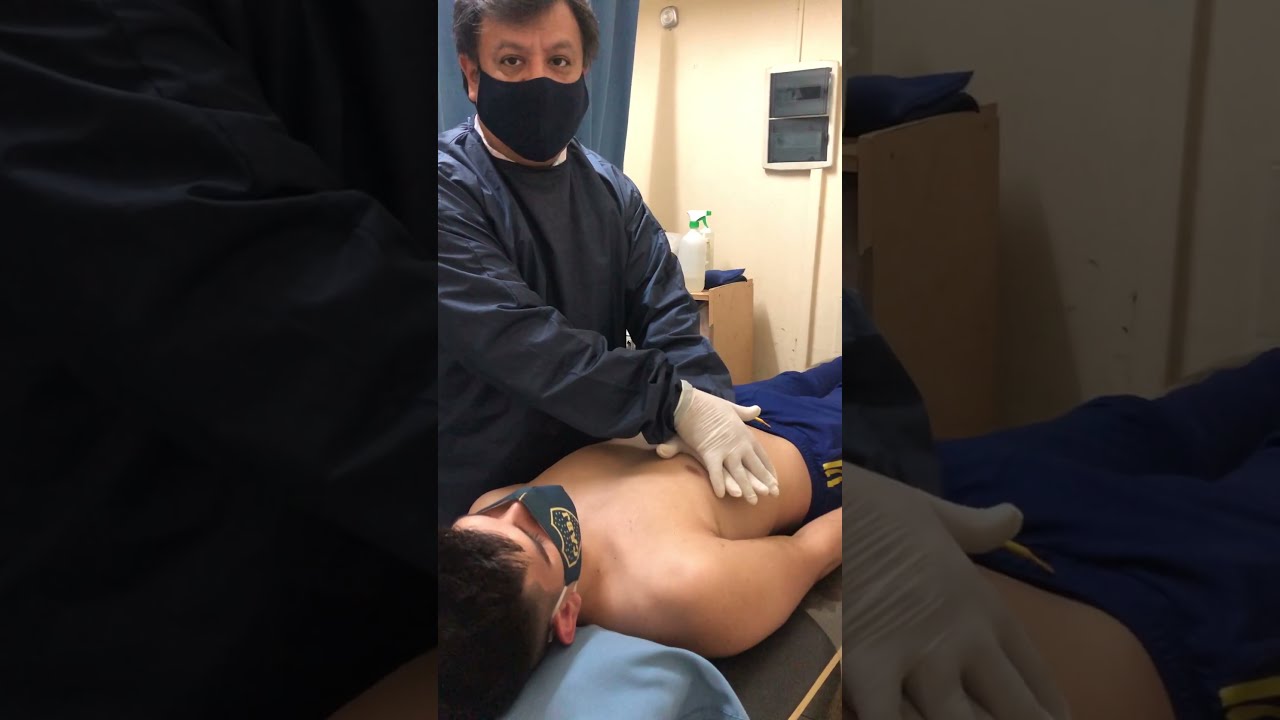The image depicts a medical scene broken into three parts: a central photo flanked by two close-up shots. In the center, a man lies shirtless on his back, wearing only blue shorts with a yellow string, and a green face mask emblazoned with yellow letters "CABJ." Attending to him is an older doctor, possibly in his 50s or 60s, identifiable by his long-sleeve navy blue surgical scrubs, white latex gloves, and a black face mask covering his nose and mouth. Both men have brown hair. The setting appears to be a brightly lit room with a blue curtain serving as a backdrop, giving a makeshift impression rather than a traditional medical facility. Behind them, there's a small wooden table holding a green and white spray bottle. The side photos offer detailed close-ups: one focuses on the doctor’s gloved hand and the patient's shorts, while the other highlights the table, spray bottle, and part of the doctor's attire. The image is clear and high-quality, emphasizing the meticulous details of the scene.